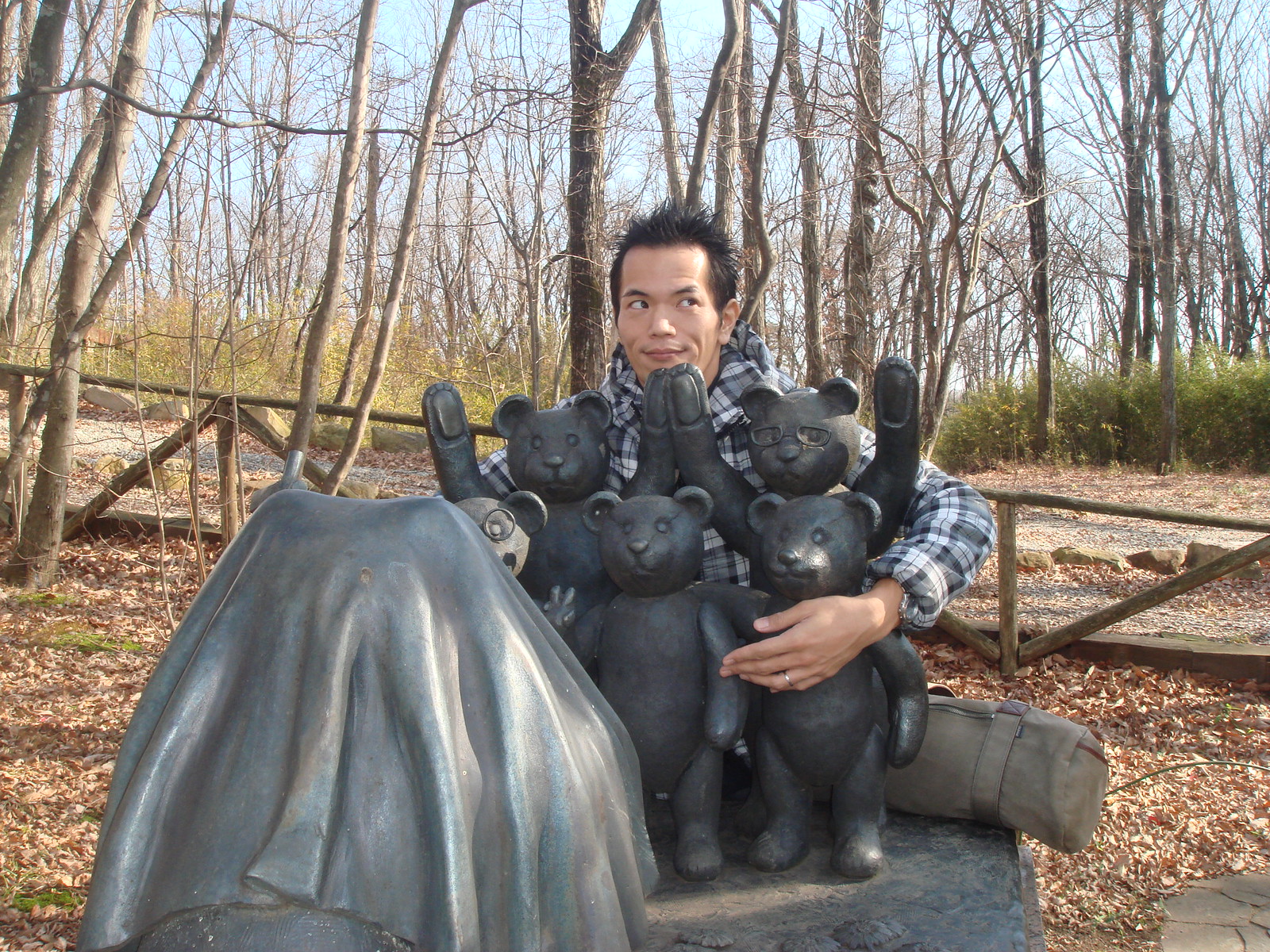In this autumnal scene set in a forested area with tall, thin, and leafless trees, a man with spiky black hair, tan skin, and wearing a blue plaid shirt is posing for a photo. He is hugging a whimsical statue of a bear family perched on a rock. The bear family consists of a dad, a mom with glasses, and three cubs, with two of the larger bears at the back raising their arms. The man, making a slightly goofy face, looks coyly off to the right. The ground around them is covered in brown leaves, though patches of green grass peek through. A wooden fence extends diagonally in the background, and the scene is lit by the clear blue sky of a sunny day, casting a few shadows. Near the man, a camping bag lies on the ground. The overall atmosphere suggests a serene and playful moment captured in a crisp, autumn day.